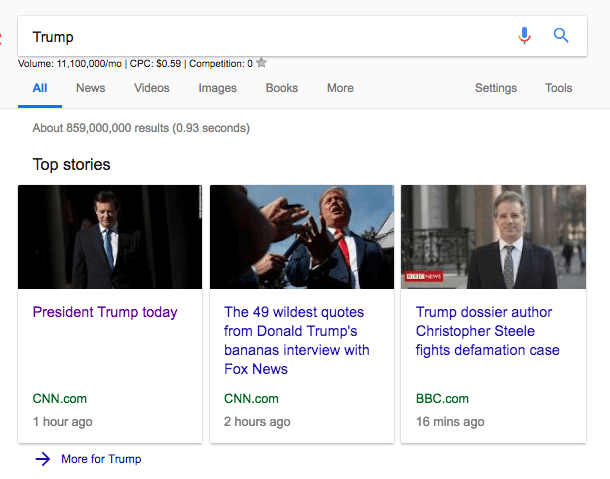The image depicts a screen capture of Google search results for "Trump." Although the Google logo is not visible, the search bar at the top shows the query "Trump." Under the search bar, the "All" tab is highlighted in blue and underlined. Below this, the "Top Stories" section is displayed, featuring three distinct news snippets:

1. The first box has a headline titled "President Trump Today," marked in purple text. It includes an image of a man with dark hair in a black suit standing in front of a curtain; however, the individual is not Donald Trump. The source is labeled as CNN.com in green, with a timestamp of "1 hour ago" in gray.

2. The middle box displays an image of Donald Trump wearing a blue suit, red tie, and white shirt. Trump is positioned on the right side of the image, seemingly in conversation with an unseen person on the left who is holding a pen, suggesting they might be a reporter. The headline reads, "The 49 wildest quotes from Donald Trump's bananas interview with Fox News," in blue text. The source is again noted as CNN.com in green, with "2 hours ago" in gray beneath it.

3. The third box features an image of a middle-aged man in a dark suit, gray tie, and white shirt, standing in front of a building with a sidewalk and people walking in the background. This man is not Donald Trump but is identified in the headline as "Trump dossier author Christopher Steele fights defamation case." The source is indicated as BBC.com in green, with "16 minutes ago" in gray.

At the bottom left corner of the screen, outside of the boxes, there's a right arrow labeled "More for Trump," which suggests an option to view additional stories.